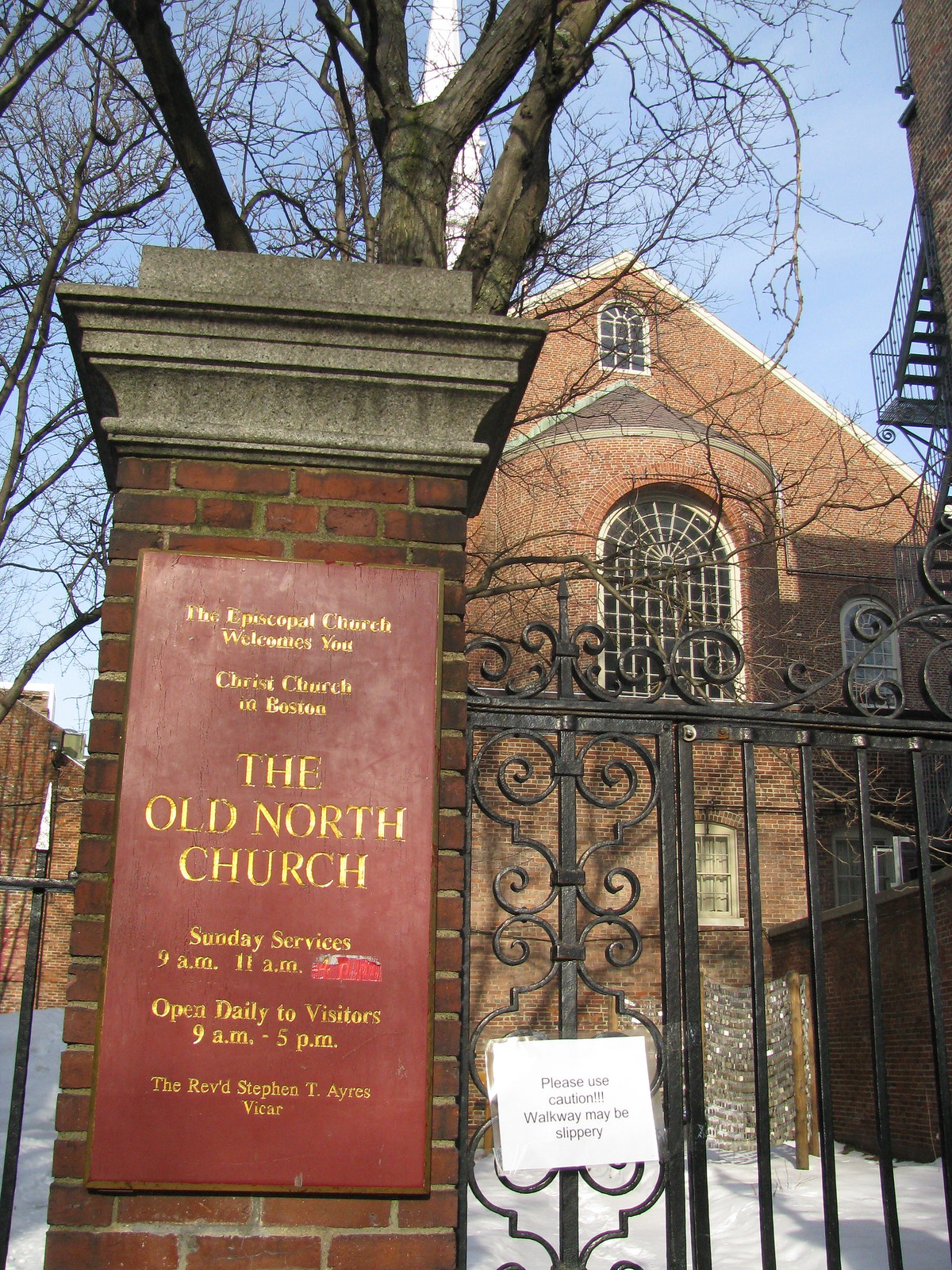The image captures the front of the historic Old North Church in Boston on a bright, clear winter's day, with a vivid blue sky and snow blanketing the ground. The central focus is the metal black fence adorned with intricate curly decorations, which stands before the church. Attached to the gate is a white sign cautioning about the potentially slippery walkway. Dominating the foreground is a prominent red sign that reads “The Episcopal Church Welcomes You, Christ Church in Boston, The Old North Church.” It details service hours, stating Sunday services are at 9 a.m. and 11 a.m., and the church is open daily to visitors from 9 a.m. to 5 p.m. Below this, it notes the Reverend Stephen T. Ayers as the vicar. Behind the gate, the church building's facade is visible, featuring a large, rounded window with multiple panes and a towering spire above. The scene is framed by a bare-branched tree, adding to the winter atmosphere. Despite its closed gates, the church invites community and visitors, blending historic charm with its seasonal setting.